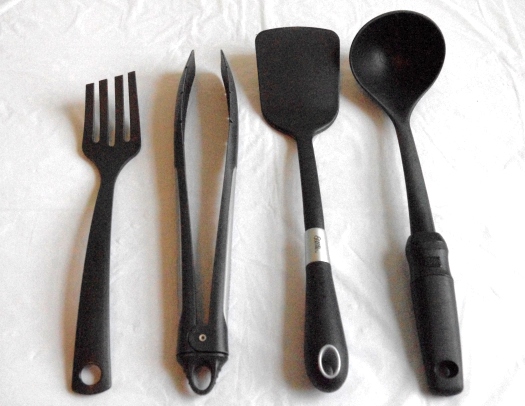The image displays four black plastic cooking utensils carefully arranged on a slightly wrinkled white tablecloth, which serves as a plain background. From left to right, the utensils are positioned in ascending order of size: a distinctive fork, a pair of tongs, a spatula, and a ladle. The fork, on the far left, features slanted prongs that progressively increase in size from left to right. Next to it are the black tongs, followed by a black spatula with a small white wraparound near its handle, and finally, the longest utensil, a black spoon-type ladle. Each utensil has either a hole or feature for hanging and they generally look like they match, although they may or may not be part of the same set.